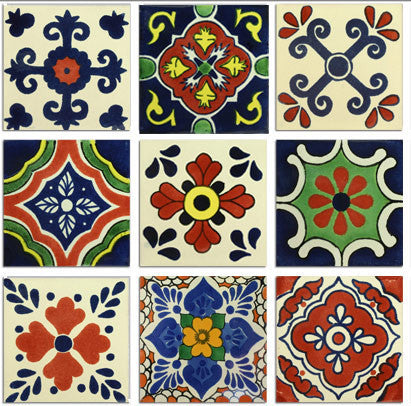The detailed image is a three-by-three grid of ceramic tiles, each measuring about three-quarters of an inch on all sides, separated by white lines. At the top of the grid is a horizontal black pinstripe border.

In the first row:
1. The top left tile has a light tan background featuring a blue and red cross-like design adorned with floral elements.
2. The top middle tile has a black background with a central red beveled diamond containing yellow accents, surrounded by green and yellow patterns.
3. The top right tile displays a light tan background with a blue X-shaped design with curls at the ends and red floral elements at the corners.

In the second row:
4. The middle left tile, has blue diamond-like background with white leaves in the center, framed by layers of white, red, green, and yellow details.
5. The center tile features a light tan background with a central black circle bordered by yellow, with red and black leaf patterns extending from the center in the four cardinal directions.
6. The middle right tile has a centralized black circle with red petals on a green background, accented with white hues along the edges and outlined in black.

In the third row:
7. The bottom left tile has a black circle with four spade-shaped leaves forming a cross-like pattern against a tan background.
8. The bottom middle tile displays a yellow flower in the center, set within a green square with surrounding blue petals.
9. The bottom right tile has a red central circle, layered with a series of black and white outlining circles, and bordered by ovals and bubble-shaped diamonds in red and black.

Each tile presents a unique combination of geometric and floral motifs, contributing to a vivid and intricate overall design.